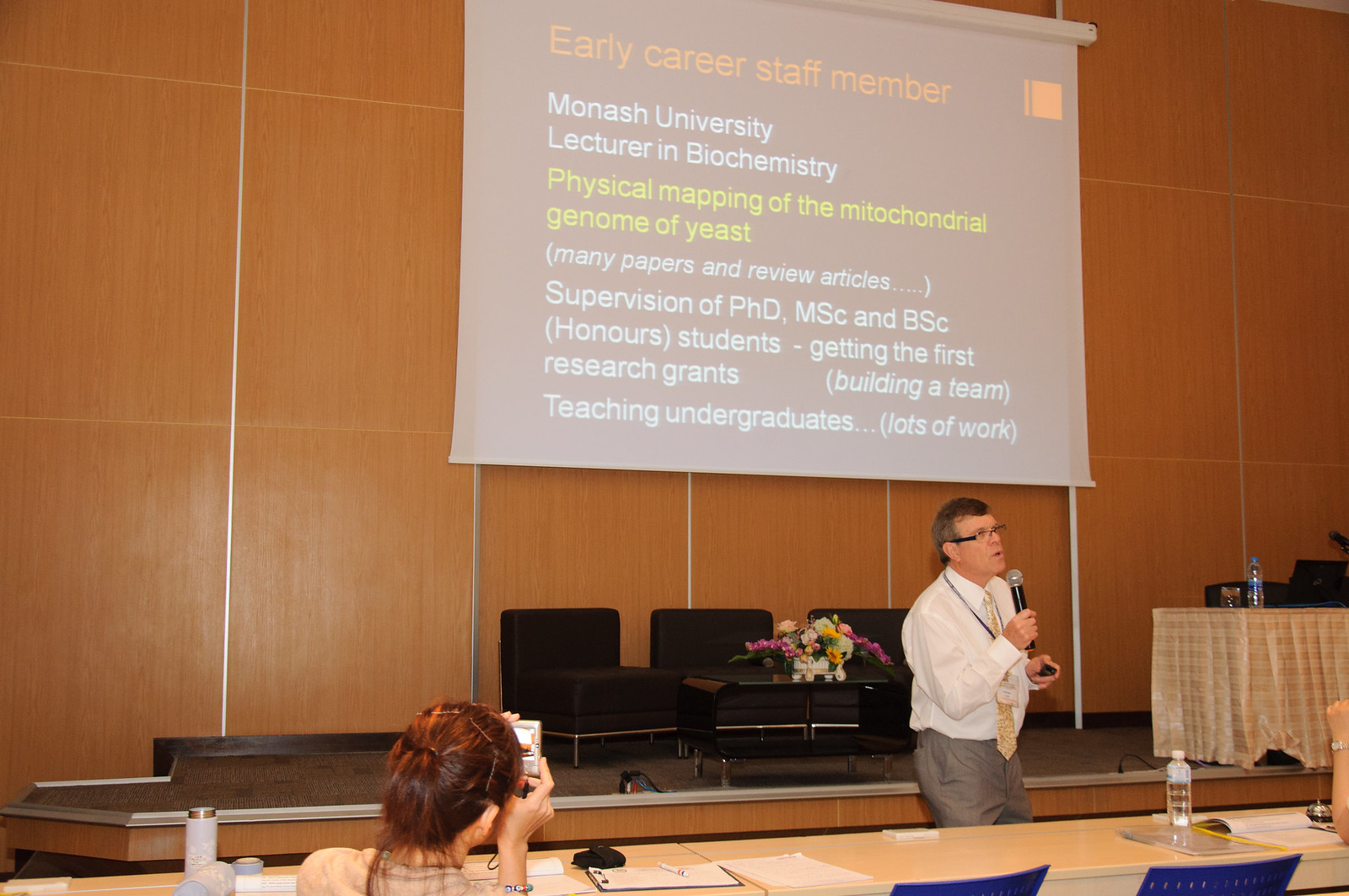In this image, a male speaker stands at the front of a room, delivering a presentation. He has short hair, wears glasses, and is dressed in a white shirt paired with very light brown or gray pants. Completing his attire, he sports a tie and a lanyard around his neck. Positioned towards the bottom right of the image, he holds a microphone, with a screen pulled down behind him displaying his presentation slide. The slide prominently reads "Early Career Staff Member, Monash University Lecturer in Biochemistry" and includes points such as "Physical Mapping of the Mitochondrial Genome of Yeast," "Many Papers and Review Articles," "Supervision of PhD, MSc, and ESC Honors Students," "Getting the First Research Grants," "Building a Team," and "Teaching Undergraduates." The text is mainly in white, with the title in orange and the phrase "Physical Mapping" highlighted in yellow. 

In the foreground, a single female attendee, seated at a table with blue chairs, watches the speaker attentively, possibly taking a photo. Behind the speaker, there is a platform with a table adorned with flowers and some chairs. Additionally, the arm of another person is partially visible on the lower right side of the image.